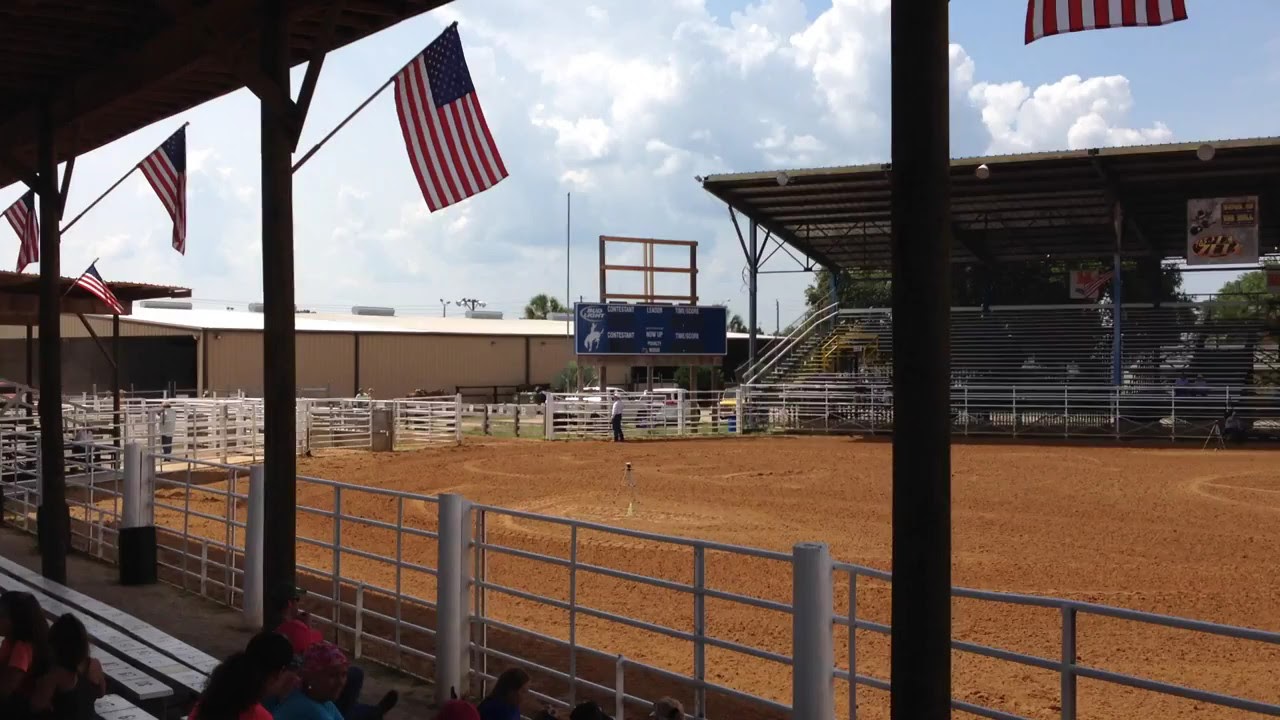This photograph captures an outdoor rodeo stadium taken during the daytime. The venue, typical for bull and bronco events commonly found in Western, middle American towns, features leveled, rich brown dirt in the arena, visibly marked by tractor treads. The arena is encircled by white metal fencing, interrupted by gates on the far left. We are sitting underneath a metal overhang designed to shield spectators from the heat, featuring vertical poles adorned with American flags. The opposite bleachers, which are mostly empty, mirror this setup. A blue stadium scoreboard, not currently lit, stands above the fence, displaying the image of a cowboy riding a horse with a Bud Light logo on top. The background reveals a striking blue sky, filled with large, thick white clouds, contributing to the picturesque setting. On the left side of the photograph, the lower bleachers where we are seated have some spectators, unlike the more vacant right side. No one occupies the rodeo field, save for one individual near the fence. Visible in the distance is a large farm building, emphasizing the rural charm of the venue.